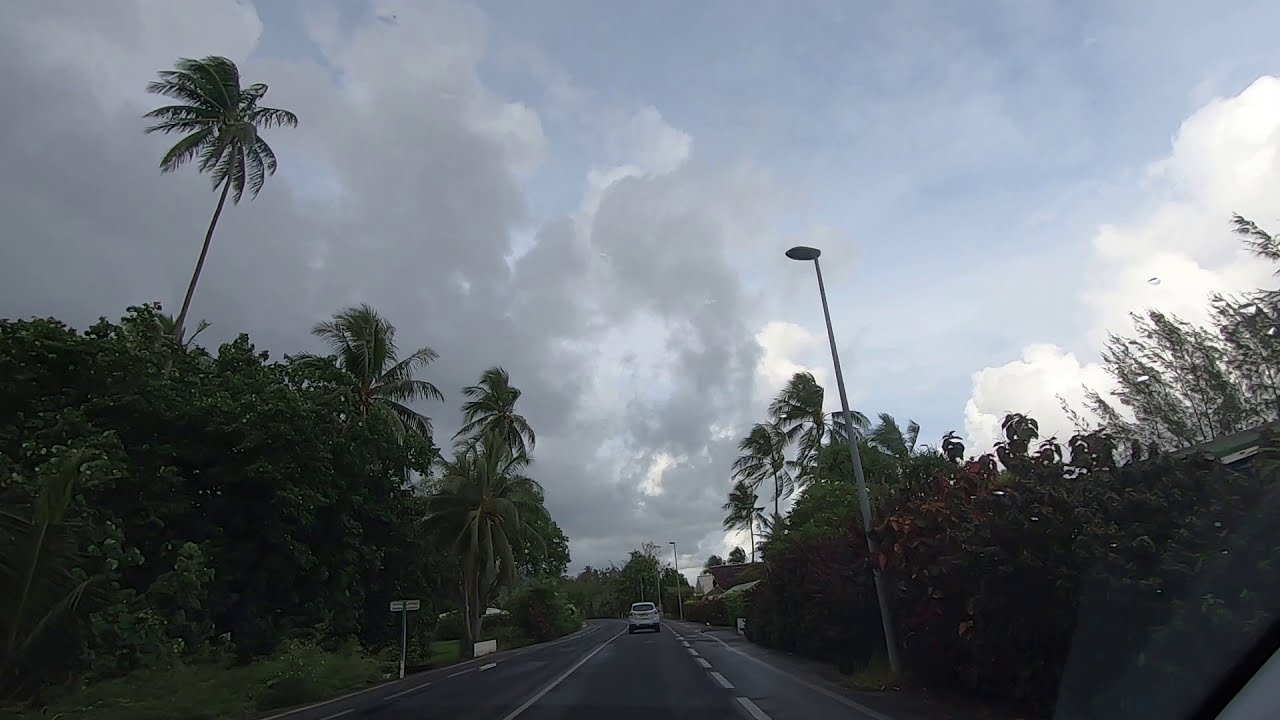The image depicts a two-lane road flanked by tall, stately palm trees, emblematic of a tropical or coastal setting. The road is marked by a solid white line in the middle and dotted white lines on each side. A white SUV, or possibly a family car, is traveling in the right lane. To the right of this vehicle, a tall lamppost stands, while further ahead on the right side of the road, a white and brown house or building is visible. The scene includes additional greenery and other smaller foliage interspersed with the palm trees. Although gray clouds dominate the sky, there are patches of blue visible, suggesting a break in the otherwise overcast weather. No pedestrians are visible, hinting at a tranquil moment captured during the daytime, likely with some wind blowing from the right side of the image to the left.